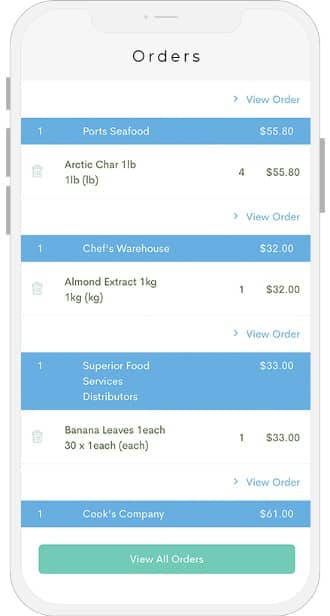The image displays a cell phone screen showcasing a list of orders within a web-based application. The interface primarily features a white background interspersed with alternating blue rectangles spanning the width of the screen. 

At the top of the screen, under the header, the first order is from **One Ports Seafood**, totaling **$55.80**. This entry details the purchase of **Arctic Char (One Pound)** with a quantity of **four**, amounting to **$55.80**, and includes a "View Order" button.

Continuing downward, the next order is from **Chef's Warehouse** for **$32**. This order specifies **Almond Extract (One KG)** with a quantity of **one**, priced at **$32**, accompanied by a "View Order" button.

The final listed order is from **Superior Food Services Distributors**, totaling **$33**. This entry notes the purchase of **Banana Leaves (Teach 30 times one each)**, with a singular quantity priced at **$33**. Each order entry includes a trash can icon on the left for removing items.

At the bottom of the screen, a button labeled "View All Orders" is visible, providing an option to review all placed orders.

The layout and detailed textual content of each entry alongside interactive elements depict a practical ordering system geared towards food and ingredient purchases.